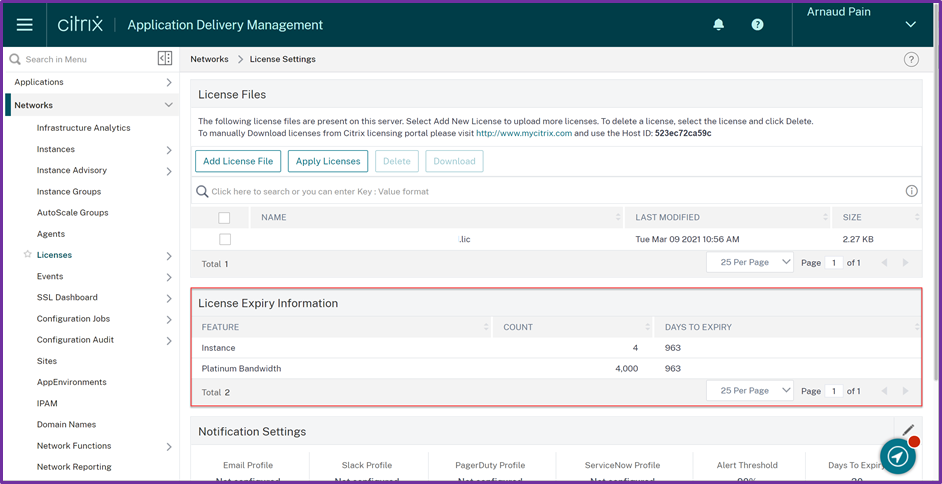The image depicts a user interface with various outlined elements and text descriptions. At the top, a purple-outlined rectangle contains a dark green rectangle. On the left side, three stacked lines in a whitish or lighter green color are present. Below this, the text "Citrix Application Delivery Management" is displayed. On the right side, there is a circular bell icon (possibly with a question mark or unreadable text) and a downward-pointing arrow beside it. Underneath, a magnifying glass icon is accompanied by some small, unreadable text. 

A tan rectangle labeled "Networks" with a right-pointing arrow comes next, potentially followed by "License Settings." Beneath this section, the label "Applications" appears. Under "Applications," "Networks" is listed again with an open green bar showing multiple networks arranged vertically. To the right, "License Files" is indicated in a light gray rectangle with additional subtext in black and green.

Several outlined rectangles follow: a green-outlined rectangle labeled "Add License File" in green, another green-outlined rectangle labeled "Apply License," and a gray-outlined rectangle that likely says "Delete." Another gray-outlined rectangle labeled "Download" is next. Near these, a magnifying glass icon is present alongside unreadable text.

In a larger gray rectangle with a white square, the columns "Name," "Last Licensed," and "Size" are noted. Below this is a white rectangle containing a gray-outlined square with an unreadable symbol and text. Further down, a sequence of gray and white rectangles with unreadable text is visible.

Highlighted in red is a rectangle labeled "License EXPIRY Information," with gray and white boxes containing tiny, unreadable text below it. Finally, a light gray rectangle labeled "Notification Settings" appears, accompanied by a green circle with an outlined white circle and an upward-right arrow. A red dot is also present near this section.